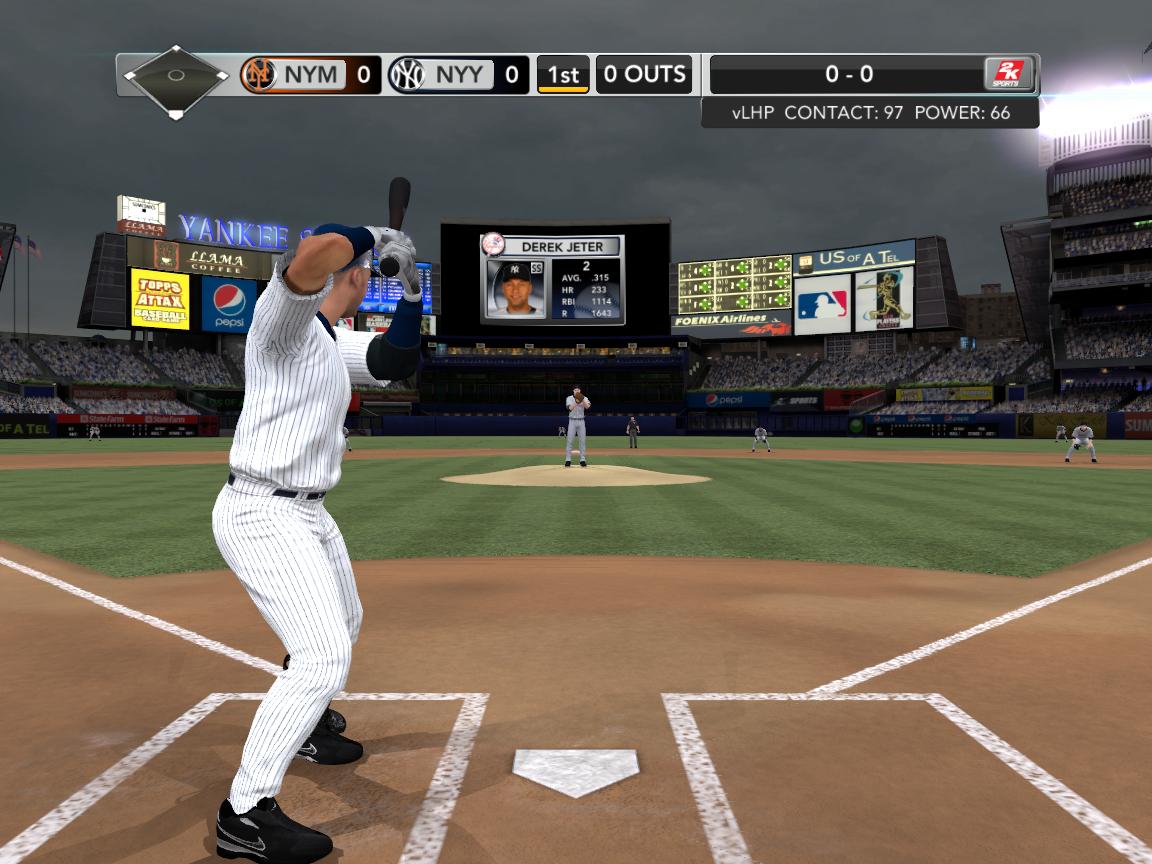The image captures an intense moment from a realistic-style baseball video game, shot from the perspective of the catcher. Centered in the frame is a batter, dressed in a uniform with black stripes, a dark blue undershirt, black arm pads, and a dark blue helmet. His black baseball bat is poised for a swing, reflecting the tension of the impending pitch. The batter stands in a brown dirt batter's box outlined with a white border, casting a clear shadow.

Ahead, the pitcher on the tan-colored mound is poised to throw, dressed in gray with a small dark blue cap and a brown glove. The field features meticulously detailed chalk lines marking the bases and the diamond layout. In the distance, several players in gray uniforms occupy their positions on the expansive green field.

The bustling stadium in the background is filled with a large crowd, and above the stands, numerous lit-up billboards and display screens feature player stats, advertisements, and team scores. Prominently displayed is Derek Jeter's name and statistics, alongside details of the ongoing game: New York Mets 0, New York Yankees 0, with zero outs in the first inning. The interface also shows advanced player metrics from 2K Sports, enhancing the immersive experience of this detailed, virtual baseball environment.